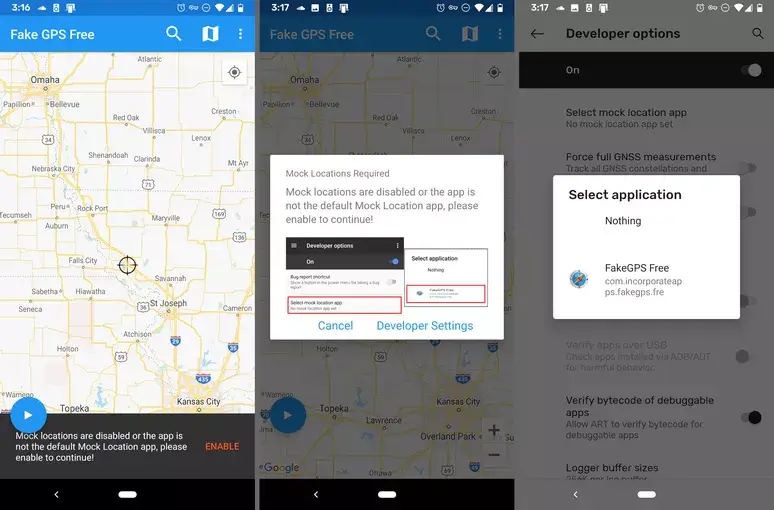The image depicts a smartphone screen with a focus on a mobile application in development. The layout consists of three rectangles arranged side by side, where the first rectangle is illuminated while the other two remain dark. This suggests ongoing development or testing activities.

In the first rectangle, the screen displays a dark blue status bar at the top, indicating the time as 3:16. Various icons are present: an alarm icon, a Wi-Fi signal symbol, and a battery icon showing three-quarters full. Below this is another graphical element inside a rectangle labeled "Fake GPS Free," characterized by a magnifying glass icon, an icon resembling a folded map, and three dot icons suggestive of a menu.

The second rectangle features a detailed map with locations such as Omaha, St. Joseph, Kansas City, and Topeka visible, indicating a geographic area around Nebraska and Kansas. Within the map, a message reads: "Mock locations are disabled or the app is not the default mock location app. Please enable to continue," accentuated by a blue circle containing a right-pointing triangle and the word "ENABLE" in orange capital letters. This message is framed by a gray rectangle. Below it lies a black rectangle with a left-pointing arrow symbol and a white oval, while a scope icon hovers between Savannah and Fall City on the map.

Further down, two grayed-out maps are present, overlain by boxes with additional instructions. The prominent text reads: "Mock locations required, mock locations are disabled, or the app is not the default mock location app. Please enable to continue." Options labeled "Cancel" and "Developer Settings" are visible, with certain areas outlined in red for emphasis, although the small text is challenging to read.

Adjacent to the above section is another box labeled "Select Application," showing "Nothing" followed by "Fake GPS Free com.incorporateapps.fakeGPS.FRE." The background mirrors the map layout initially displayed, emphasizing a continuous map theme.

The final section highlights developer options within the phone's settings, signifying the configuration and fine-tuning necessary for app development and testing.